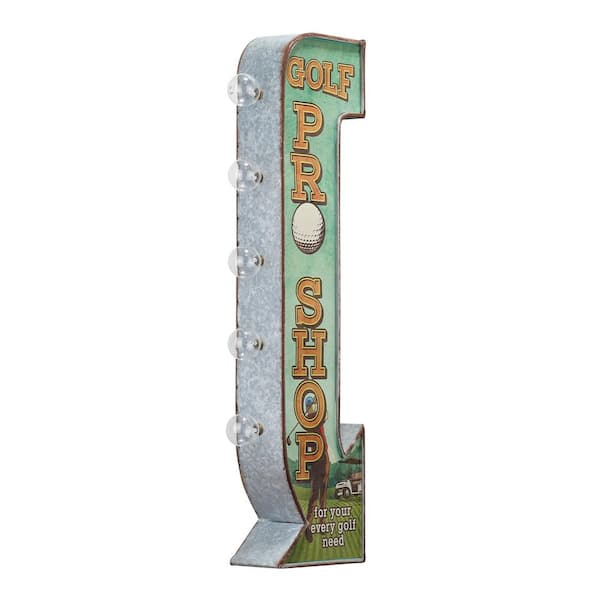This colored photograph captures a vintage metal sign for a Golf Pro Shop, designed in the shape of an arrow pointing down and slightly to the right. The sign features golden yellow text that reads "Golf Pro Shop," with the letter 'O' replaced by a white golf ball. Below this, it states "For Every Golf Need." The background of the sign is predominantly teal, transitioning to a golf-themed image near the arrowhead. This image depicts a golfer in action, a green fairway, and a golf cart in the distance. The edges of the sign are metallic, and one side is adorned with five circular lightbulbs, suggesting that the sign is illuminated at night for visibility.